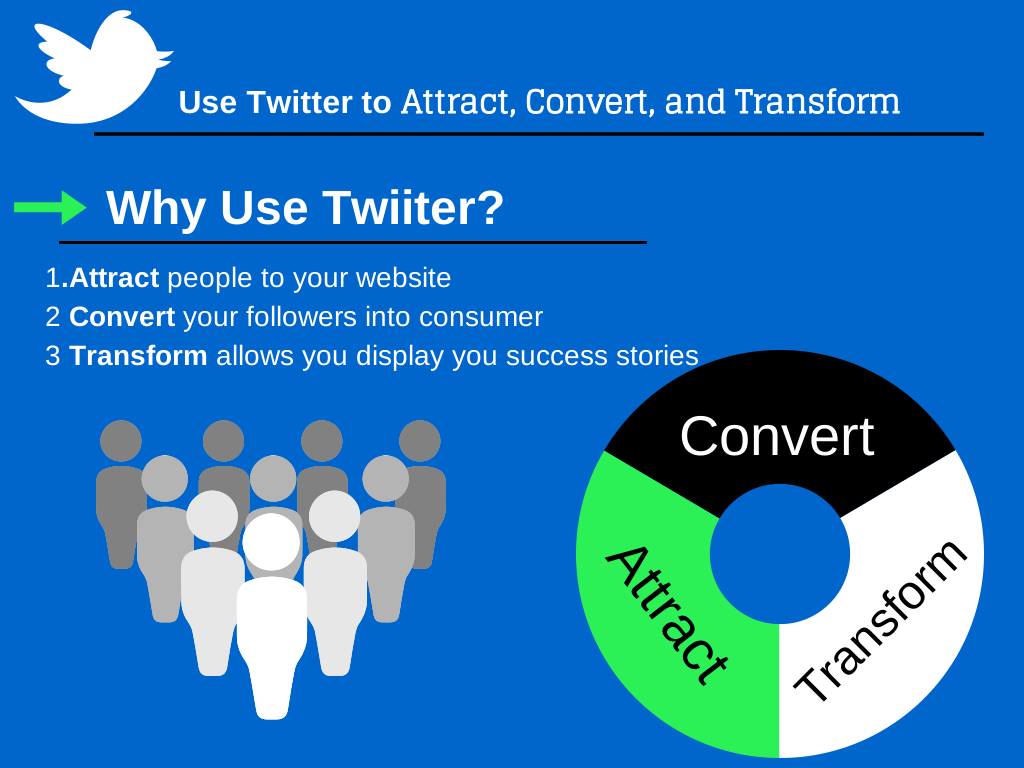A vibrant infographic with a purple background showcases a cartoonish white bird silhouette, reminiscent of the Twitter logo, in the upper left corner. The bird, depicted in profile with its wing raised, faces to the right. Adjacent to the bird, in bold white font, reads: "Use Twitter to attract, convert, and transform."

Beneath this text, a prominent black line separates the header from the rest of the content. Directly below the line, a green left-pointing arrow is accompanied by the white text: "Why use Twitter?" (notably misspelled as "Twiiter"). Following another black line, the infographic presents a numbered list:

1. Attract people to your website.
2. Convert your followers into consumers.
3. Transform allows you to display your success stories.

Towards the bottom, the image features an icon of silhouetted gray people, symbolizing an audience or user base. To the right of this icon, a circle encapsulates the words: "convert, attract, transform," reinforcing the central theme of the infographic.